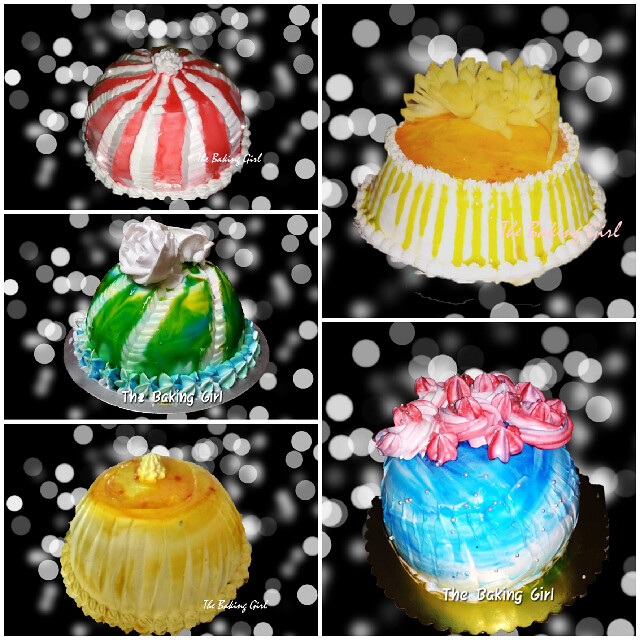This image showcases five individually designed pastries, each uniquely decorated and enclosed in a white outline. A clear line divides the image in the center, with three pastries on one side and two on the other, and additional dividing lines separating each pastry. The background is black with white and gray circle patterns resembling a lighting source. All pastries carry the text "The Baking Girl" underneath them.

In the top left corner, there's a pastry featuring red and white circular stripes with a ruffled frosting. Below it, a lime green, cylinder-shaped pastry with white stripes turns upward, adorned with white frosting on top and a blue ruffled edge. The middle pastry is light yellow with ruffled and textured sides, round in shape, and topped with a darker orange hue and a small yellow bit of frosting. In the right corner, there's a pastry with ruffled yellow frosting on top, yellow and white striped edges, and additional ruffled circular edges around both the top and bottom. Finally, the bottom right corner displays a light blue pastry with white texturing, a pink flower-shaped frosting on top, and green cylindrical edges around the bottom.